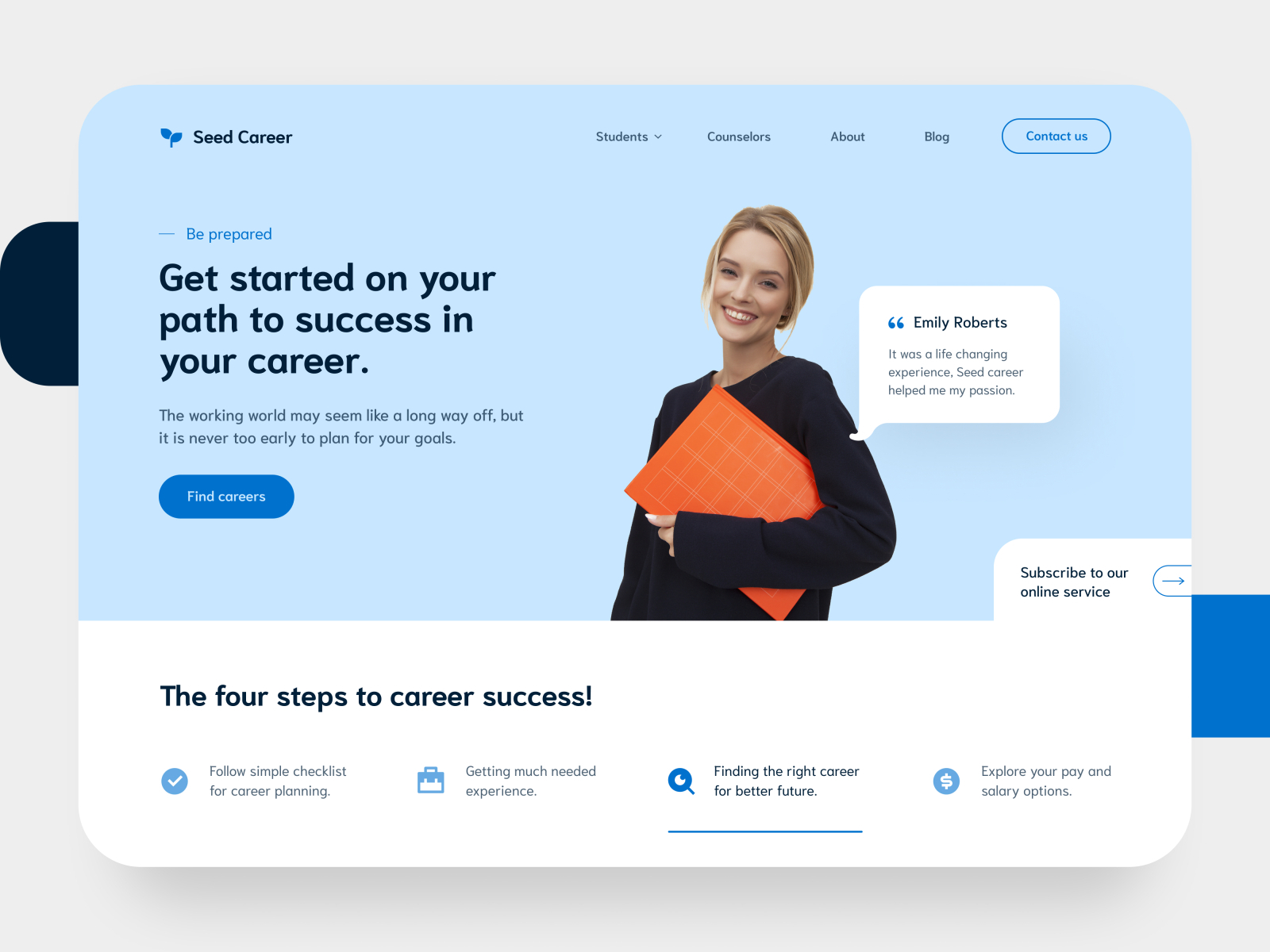In this emergency seed carrier event, students had the opportunity to connect with career counsellors, learn about blog resources, and access our "Contact Us" support. The message emphasized the importance of being prepared and encouraged students to start on their path to career success. Even though the working world might seem far off, planning early for your career goals is crucial. Participants were introduced to the four essential steps to career success:

1. Following a simple checklist for career planning.
2. Gaining much-needed experience.
3. Identifying the right career for a better future.
4. Exploring pay and salary options.

One student, Emily Robots, testified to the program's impact, saying, "It was a life-changing experience. Seed Career helped me discover my passion and set me on a path to success."